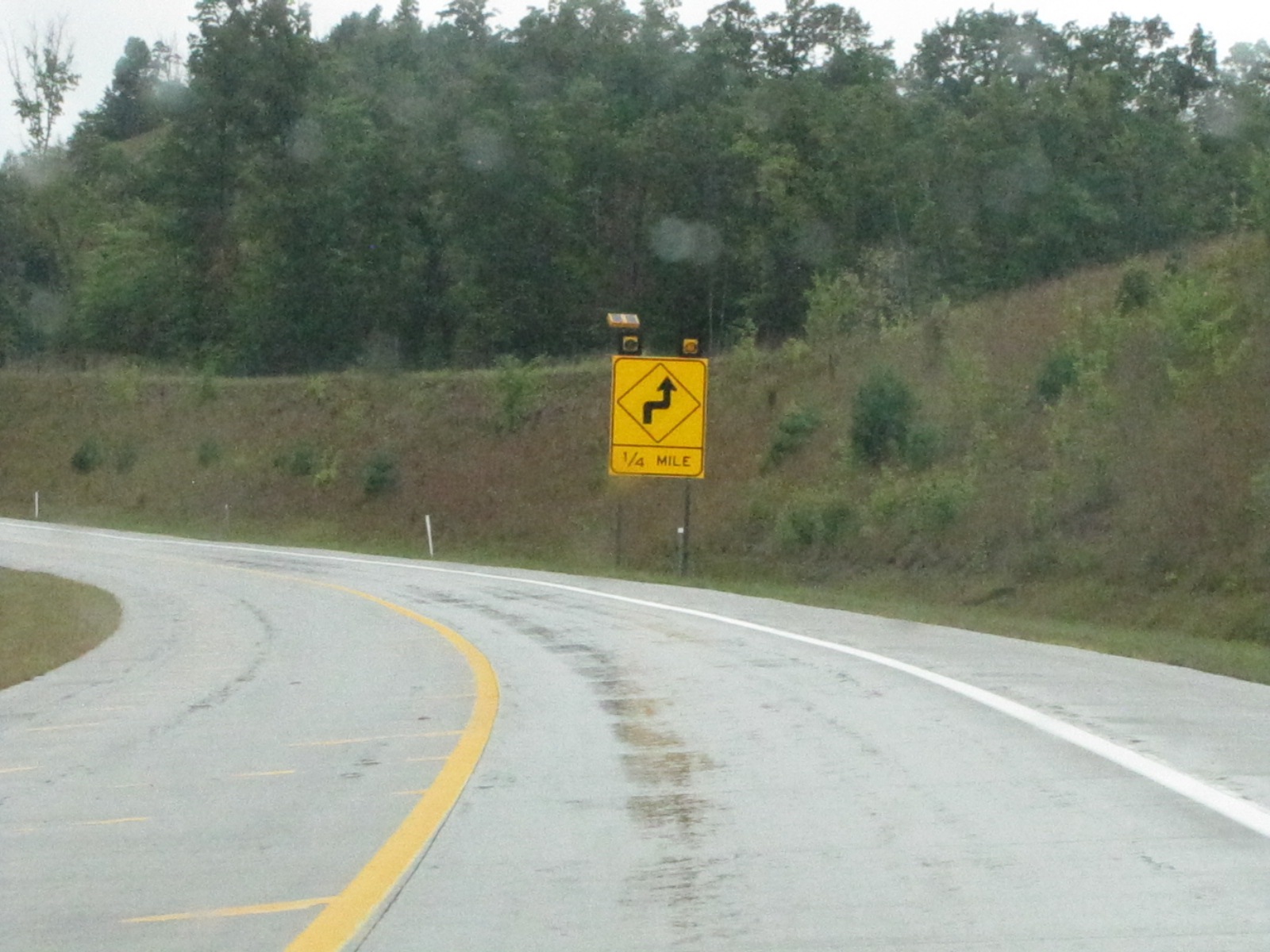This photograph captures a single-lane road bending sharply to the left, distinguished by a white stripe on the right and a yellow stripe with water droplets on the left, suggesting recent rainfall. The road, possibly an entrance or exit ramp to an interstate, follows the contour of a large hill, covered in grass and shrubs, rising alongside the curve. Atop the hill, a dense tree line stretches out under an overcast sky, enhancing the scene's moody ambiance. A prominent rectangular yellow sign bordered in black, equipped with two lights on top, stands ahead on the right side. The sign features a diamond shape with an arrow indicating a right turn followed by a straight path, accompanied by the text "¼ mile" beneath the arrow, warning motorists of the upcoming bend.